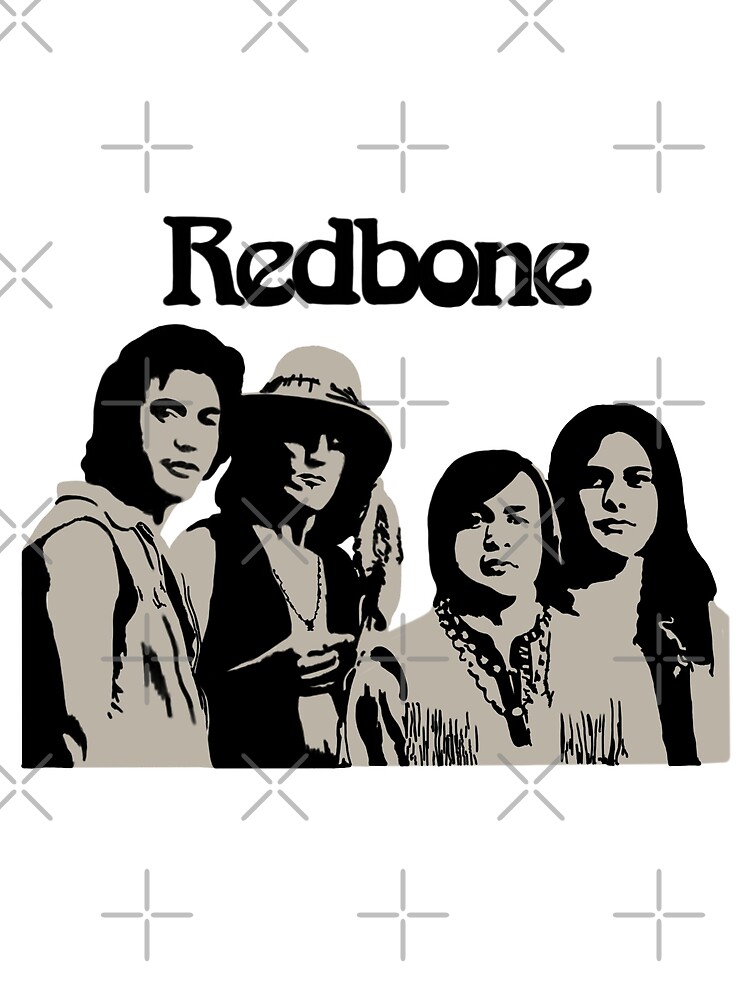The image features a digital illustration of four individuals, rendered in black and light gray on a white, empty background. The entire composition has a posterized style, characterized by large, distinct blocks of color. Overlaying the image are faint plus and X signs, possibly acting as watermarks or mockup indicators. 

At the top, bold black text reads "Redbone." The four people in the center appear to be in their 20s or 30s, dressed in a hippie style suggestive of a rock band. From left to right: the first person wears a hoodie and has long hair. Next to them is an individual in a floppy hat and a vest, also with long hair. The third person is adorned in a frilly shirt and two necklaces, with notably thick eyebrows. The fourth person has long hair. All three men are clean-shaven, while the woman, positioned inconsistently in the accounts, also has long hair.